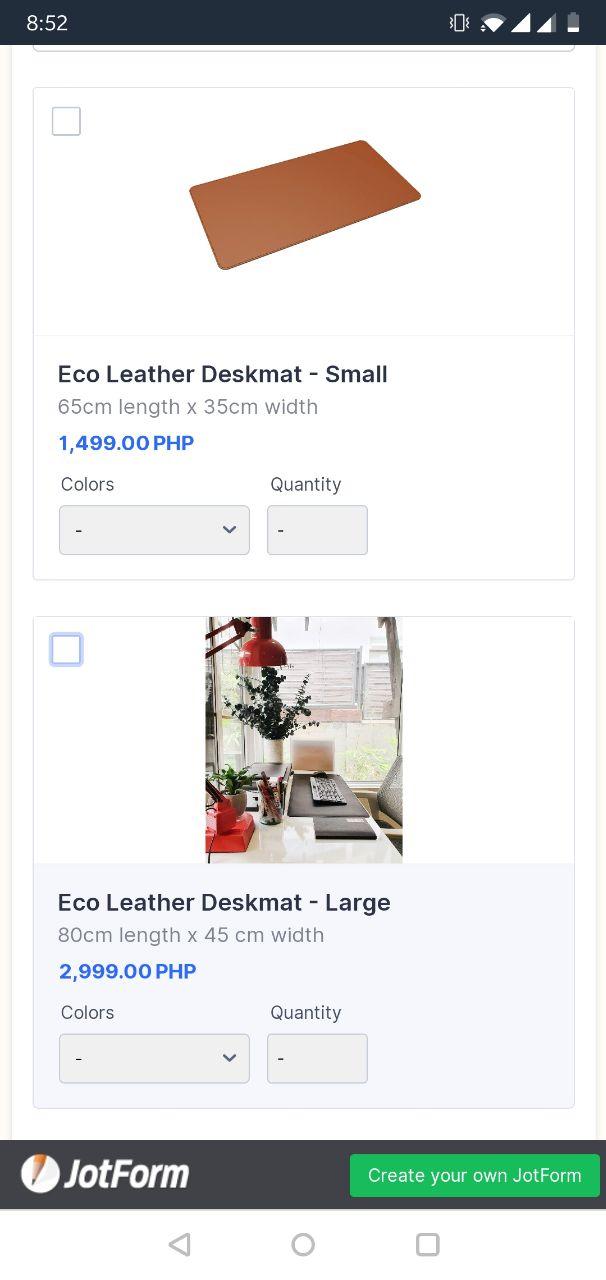This image is a screenshot taken from an iPhone, showcasing a shopping page for eco-leather desk mats. The phone’s status bar indicates that the time is 8:52, it's set to vibrate mode, has a decent signal, connected to WiFi, and the battery is approximately 30% charged.

In the screenshot, there are two product listings, each within a white box defined by a small square in the top corner.

### First Product:
- **Item**: Eco-Leather Desk Mat (Small)
- **Image Description**: A brown, leather-like desk mat.
- **Dimensions**: 65cm (L) x 35cm (W)
- **Price**: ₱14.99 PHP (approximately $15 USD)
- **Options**: Drop-down menus for selecting color and quantity.

### Second Product:
- **Item**: Eco-Leather Desk Mat (Large)
- **Image Description**: 
  - The mat is on a desk, with several items placed on top of it. 
  - Items include a black keyboard that covers the span of the mat, a tumbler filled with pencils and pens positioned behind the mat, and a composition book next to the keyboard. 
  - Additional details include a red lamp mounted higher on the wall, a red clock facing away, a larger potted plant in the corner by the windows with the blinds up, and a smaller potted plant.
- **Dimensions**: 80cm (L) x 45cm (W)
- **Price**: ₱2,999 PHP
- **Options**: Drop-down menus for selecting color and quantity.

### Footer:
- **Additional Element**: A black box at the bottom with a pencil icon, featuring the text "JotForm" and "Create your own JotForm."

This detailed description offers a comprehensive view of the products and layout of the shopping page, capturing all visual and textual information from the screenshot.